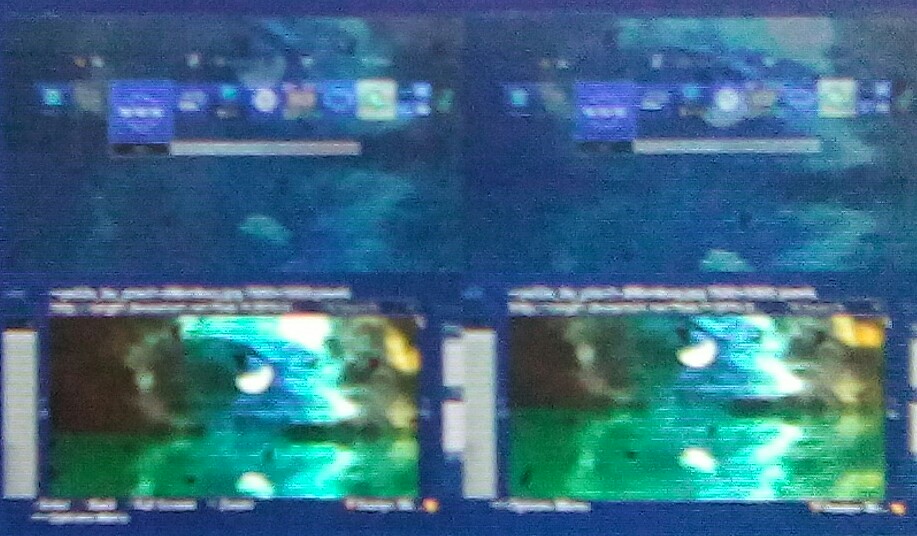This is a horizontally oriented, extremely blurry and out-of-focus image that appears to be a composite of four rectangular screenshots, arranged in two above two, creating four equal quadrants. These quadrants are displayed on a dark blue background and exhibit a dominant blue color scheme. The top two rectangles are nearly identical, featuring a row of variously sized blue and light blue squares and rectangles running just above the center. The far left square contains a circular object along with some white text. The bottom two rectangles similarly resemble each other but differ from the top pair. They feature more green and turquoise hues, possibly depicting an underwater scene with lighter greenish elements that resemble mountains and white half-moon shapes floating within. Each quadrant has white text within the margins, adding to the complexity and enigmatic nature of the blurred image.